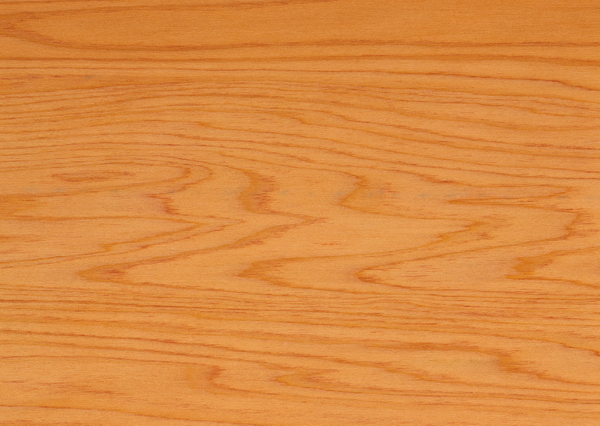The image is a detailed, color photograph in landscape orientation, focusing solely on a rectangular piece of wood. The wood, a light honey brown or light orange cream color, features a texture highlighted by its prominent grain lines. These lines, in varying shades of darker brown to brick-red, create a pattern that becomes more tightly packed near the bottom and almost at the top, while loosening in the middle and extreme top sections. The grain lines follow mostly horizontal wavy flows with zigzag patterns near the bottom half. The wood surface, devoid of any prominent knots or text, fills the entire frame, giving a realistic and representational view of its natural texture and color. The photo captures this piece of wood from a straight-on perspective, potentially as a flat wood print, with no discernible setting or time of day.